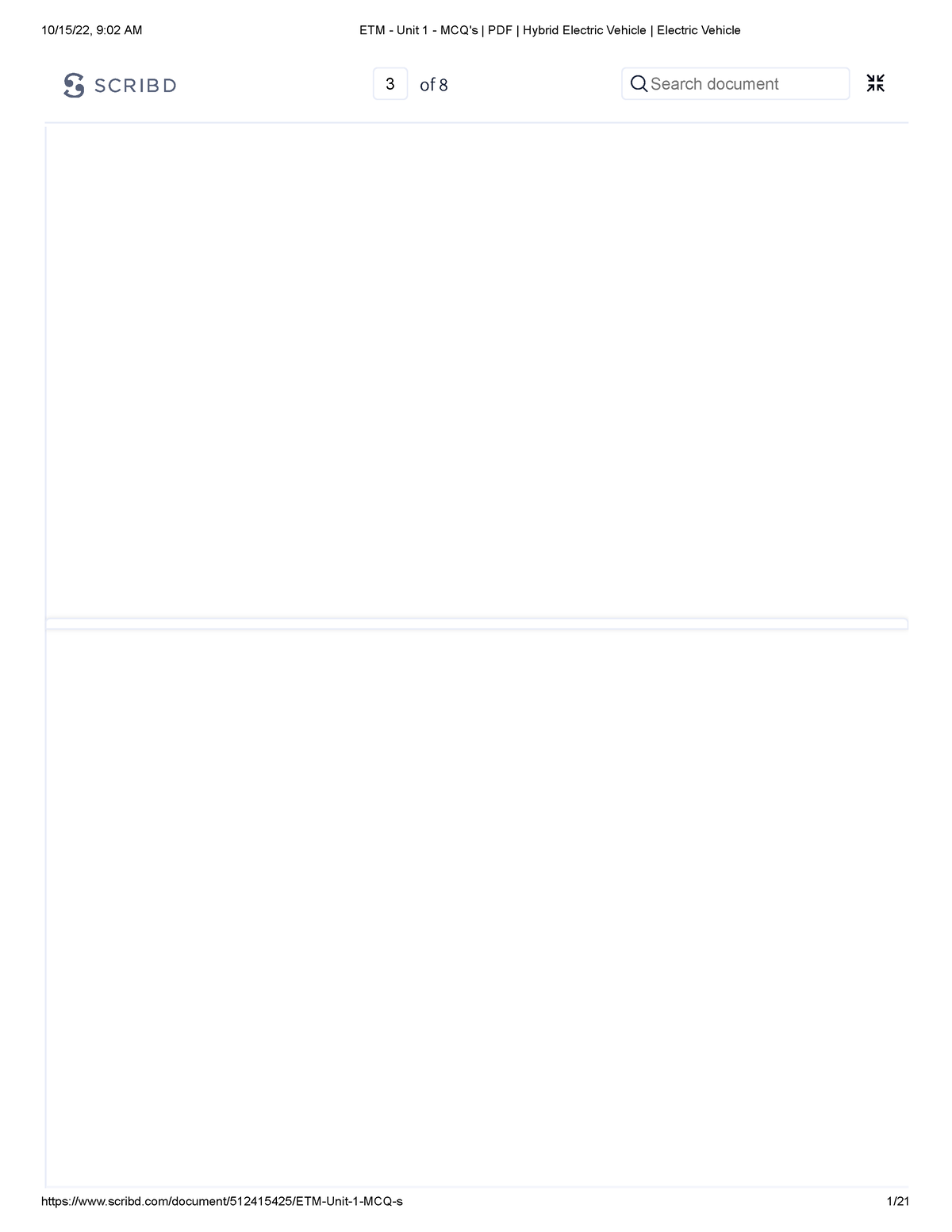This image displays a section of a webpage from the document-sharing site Scribd. The URL, visible on the bottom left of the screen, is "https://scribd.com/document," indicating an open document. On the bottom right, pagination information reveals that this is a 21-page document, although the current view shows two blank pages side by side. Oddly, the top of the screen indicates "3 of 8," suggesting that multiple pages may be condensed into a single panel or pane. The content of the pages shown is entirely blank, devoid of any writing or document information. Visible metadata includes a timestamp of October 15th, 2022, at 9:02 a.m., and the document's title: "PDF Hybrid Electric Vehicle." Therefore, the document seems to be about hybrid electric vehicles, but no specific content is presently visible.